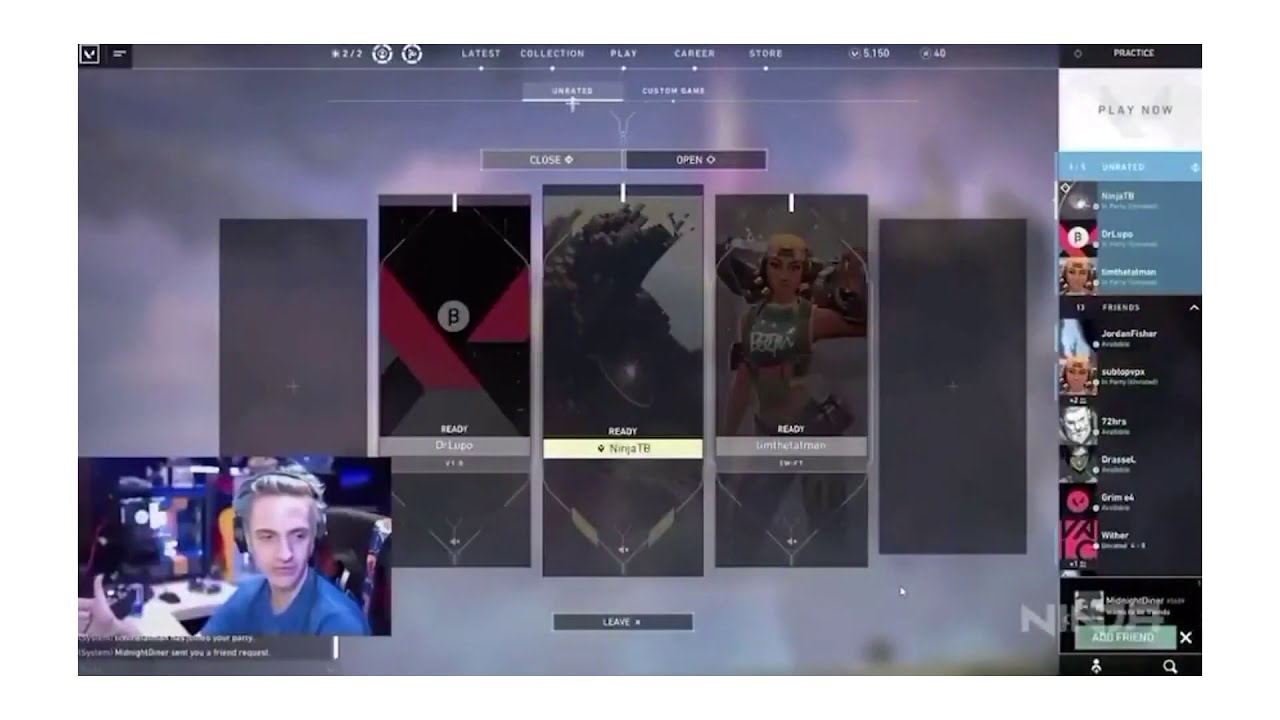In the image, we see a detailed perspective of a computer screen capturing the interface of a gaming application. At the top of the screen is a menu bar with options like "Latest," "Collection," "Play," "Career," and "Store." Centered on the screen are several rectangular cards featuring various content, likely related to different games or gaming profiles. One notable card displays a video game character adorned in a green top and yellow middle.

To the left side of the image, there is a live video feed of a streamer. This gamer, a Caucasian male with blonde hair, is wearing a blue short-sleeved t-shirt and a headset, and is seated in a black gaming chair with a white desk in front of him. He is gesturing with his hand, possibly giving a thumbs-up sign. This section, a small rectangular cutout, occupies the bottom left-hand corner of the screen.

On the right-hand side, there's a column with a white rectangular header that reads "Play Now," containing a list of gaming thumbnails or profile icons, along with some accompanying text that is too small to decipher clearly. Further down this right side, there's a list labeled "Friends," showcasing several individual profiles with options, such as adding new friends.

The overall layout is sectioned into three main parts: the top menu bar, the center area showcasing game cards and gaming profiles, and the left and right panels displaying the streamer's video feed and the friends' list, respectively.